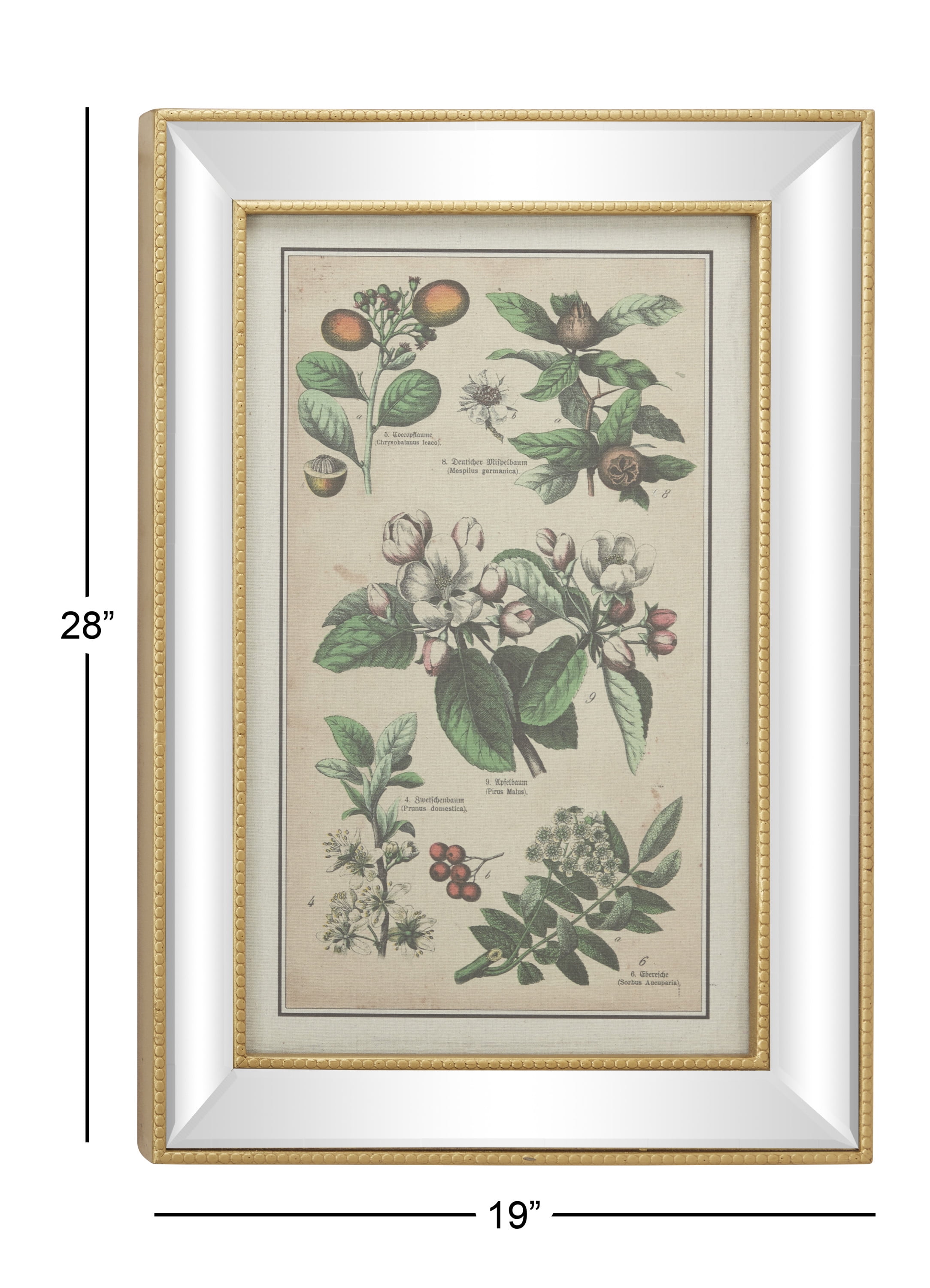This detailed illustration features a framed botanical print measuring 28 inches in height and 19 inches in width, indicated by the measurements along the left-hand side and bottom edge. The frame itself is ornate with a double gold beading pattern - one on the outer edge and one on the inner edge - separated by a white infill. The inner black matting enhances the vintage aesthetic of the print, which resembles something one might find in an antique botanical identification book or a scientific poster favored by botanists.

The artwork meticulously showcases an array of plant species, each labeled with their scientific genus and type, likely in Latin. The top section depicts three variations of flowers, including large round leaves with orange blooms on the left and pointy green leaves with grey flowers on the right. The middle section features broad leaves adorned with white and pink flowers. In the bottom section, there are delicate renderings of ferns and fruits, such as a small round fruit emerging from a sprig, along with additional flower species.

The colors throughout the print are muted, evoking a sense of aged paper, as if washed in tea, reinforcing the vintage feel. The plants are illustrated with great attention to detail, displaying green leaves, white petals, and various colors of seeds or berries, including brown, orange, and red. This comprehensive botanical illustration not only serves as a scientific record but also as a piece of aesthetic beauty, perfectly framed for display.